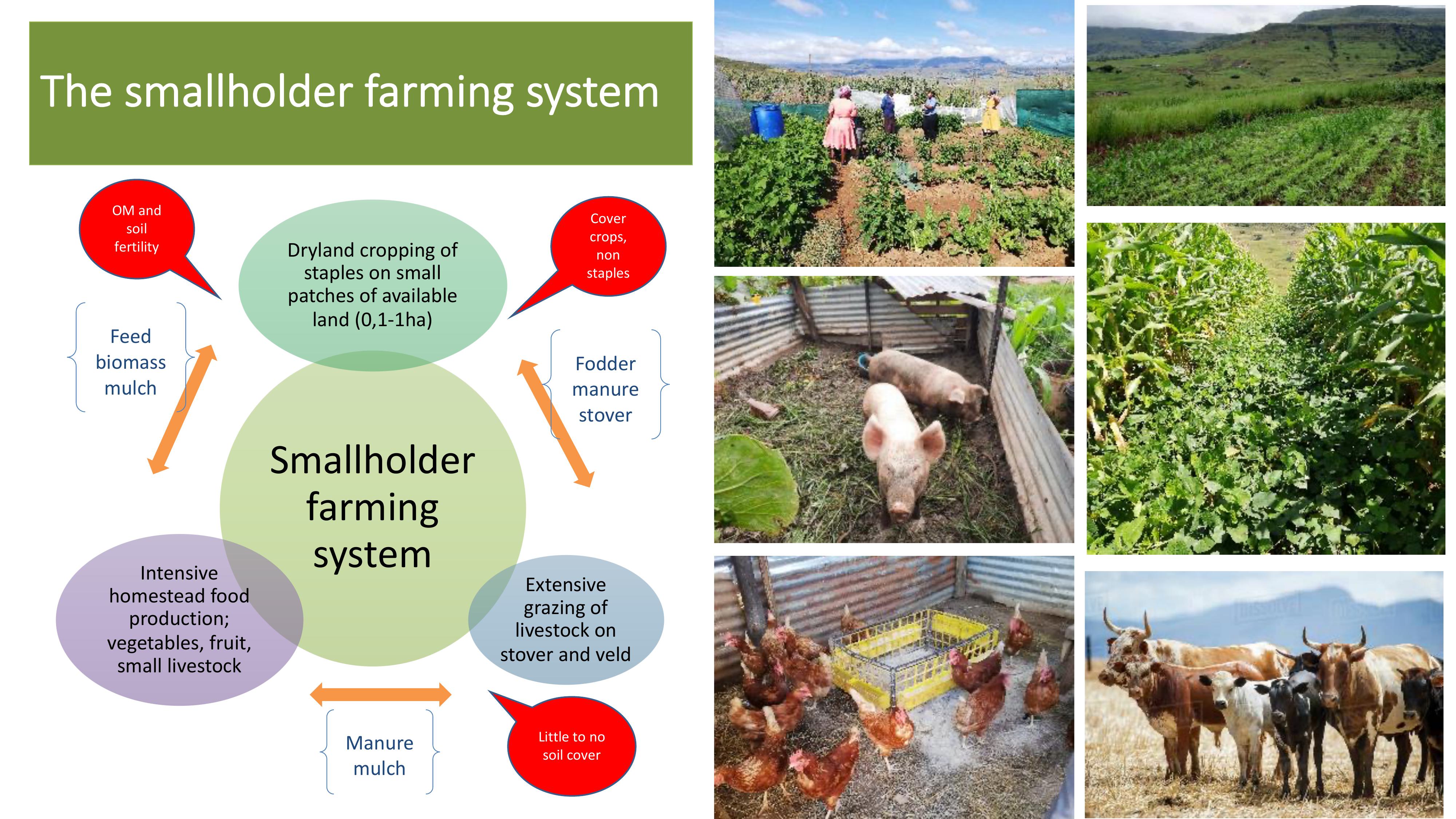The image presents a detailed overview of the Smallholder Farming System. On the left side, a section labeled "Smallholder Farming System" discusses various aspects through text bubbles. These include "Dryland cropping of staples on small patches of available land," "Intensive homestead food production: vegetables, fruits, small livestock," and "Extensive grazing of livestock on stover and veld." Other arrows from the section mention topics such as "little to no soil cover," "cover crops," "non-staples," "DM," and "soil fertility."

The right side features a series of six photographs illustrating different elements of the farming system. The top two photos showcase extensive farmlands. The middle left photo captures a group of pigs, while the adjacent middle right photo again focuses on farmlands. In the lower section, the left-hand photo displays chickens, and the right-hand photo portrays cows in a grazing area. Together, these textual and visual elements provide a comprehensive depiction of the integrated and multifaceted nature of smallholder farming.